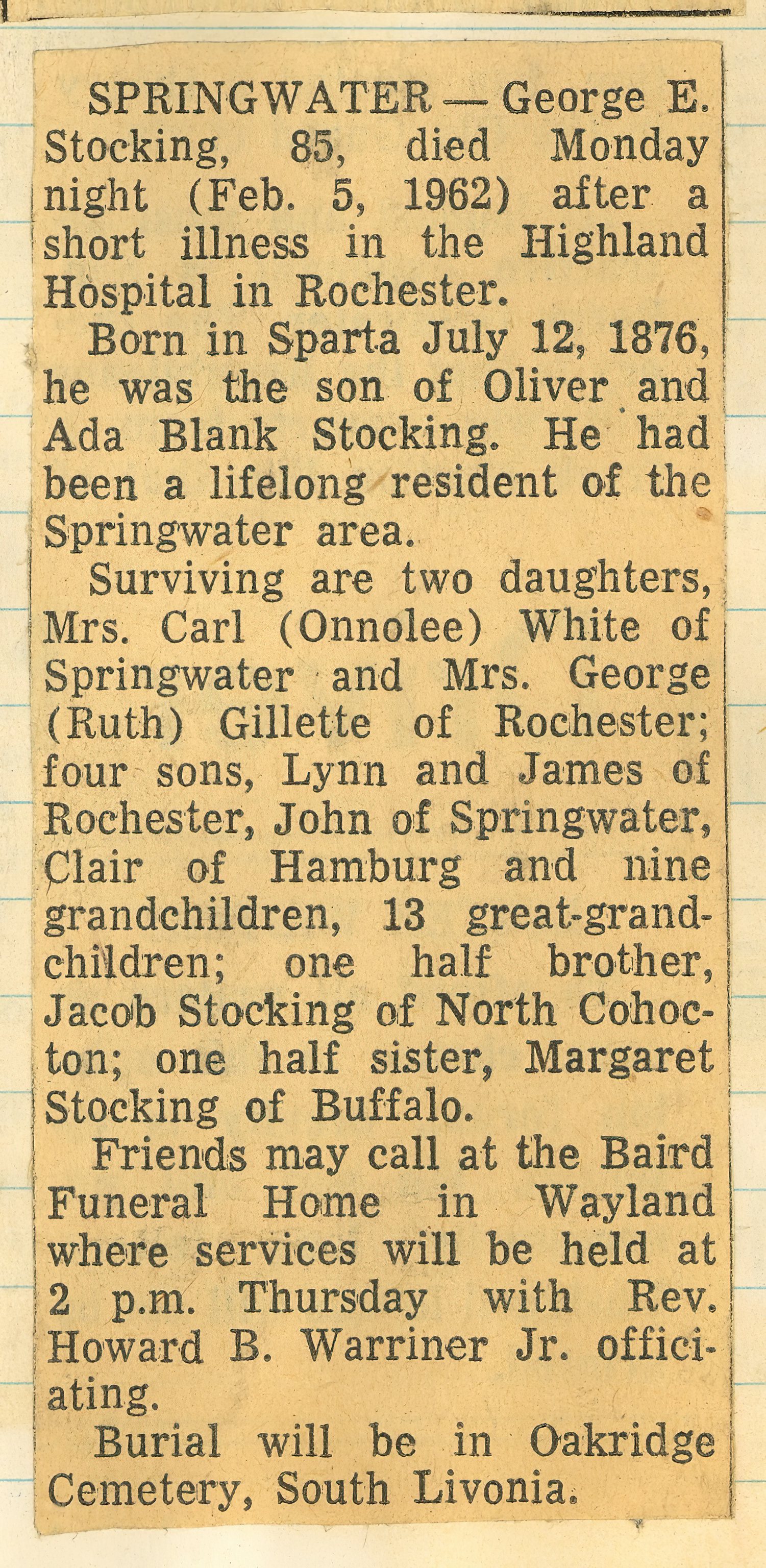This image depicts an old, yellowed newspaper clipping of an obituary, possibly from February 5, 1962, pasted onto a piece of yellow lined paper. The obituary is for George E. Stocking, a lifelong resident of the Springwater area, who passed away on Monday night at the age of 85 after a short illness in Highland Hospital, Rochester. Born in Sparta on July 12, 1876, to Oliver and Ada (Blank) Stocking, George is survived by two daughters: Mrs. Carl (Onalee) White of Springwater and Mrs. George (Ruth) Gillette of Rochester; four sons: Lynn and James, both of Rochester, John of Springwater, and Claire of Hamburg; nine grandchildren; 13 great-grandchildren; one half-brother, Jacob Stocking of North Cohockton; and one half-sister, Margaret Stocking of Buffalo. Friends can pay their respects at the Baird Funeral Home in Wayland, where a service will be held at 2 p.m. on Thursday, officiated by Reverend Howard B. Warner, Jr. Burial will follow at Oak Ridge Cemetery in South Livonia.